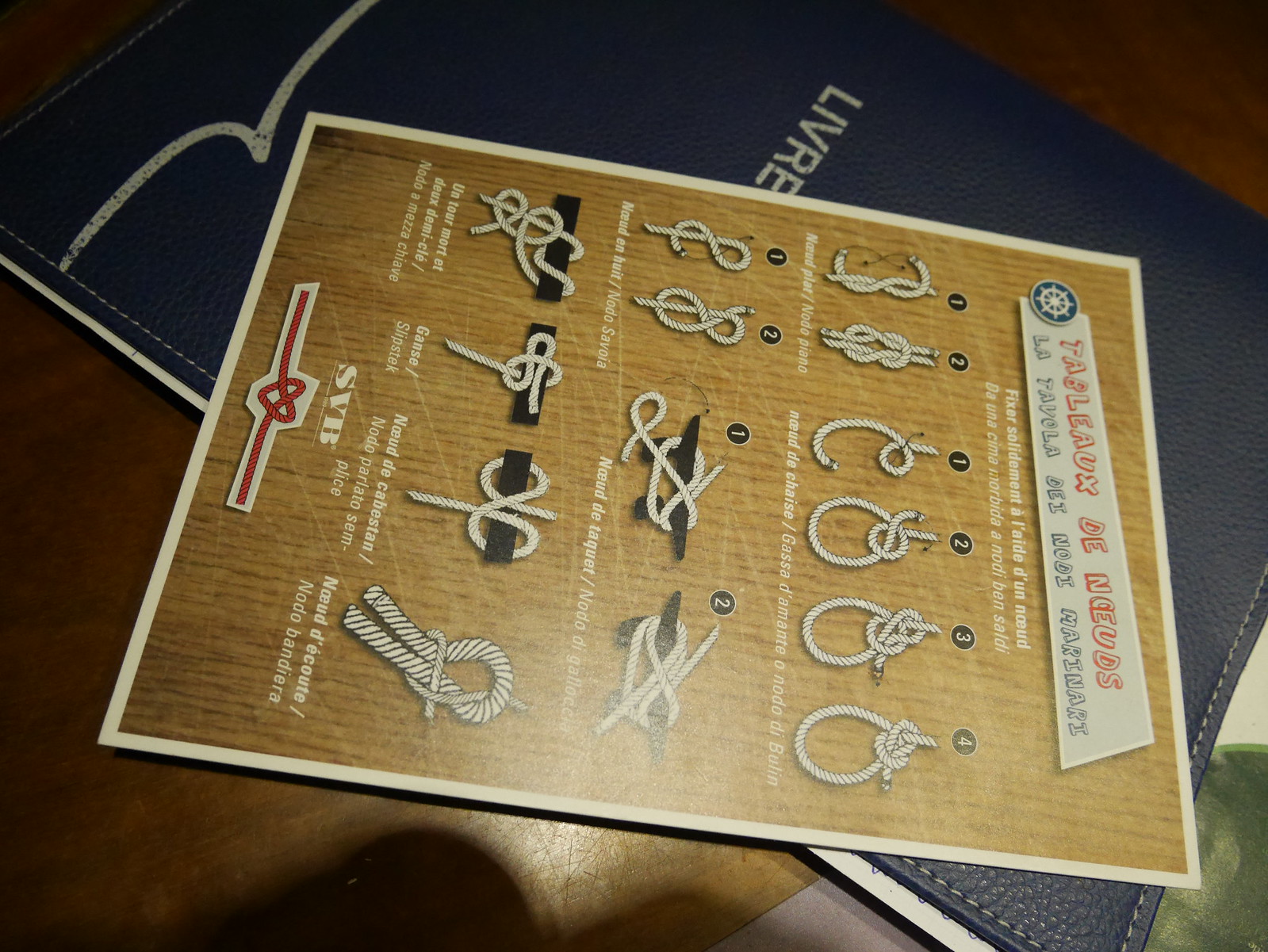This image showcases a close-up of items arranged on a dark wooden desk, revealing a partial view of the desk in the lower left, upper left, and upper right corners. Shadows cast from the bottom left corner add depth to the scene. In the lower right corner, a green element peeks into the frame. The centerpiece of the image features a black book or notebook, titled "L-I-V-R-E" in white letters, with a white squiggly line at the bottom. The book is angled almost upside down, requiring a tilt of the head to read. Positioned on top of the black book is a brown sign or pamphlet illustrating various rope-tying knots, written in French. Additionally, there is a piece of paper with step-by-step knot-tying instructions, also in French, lying on what appears to be a blue folder.